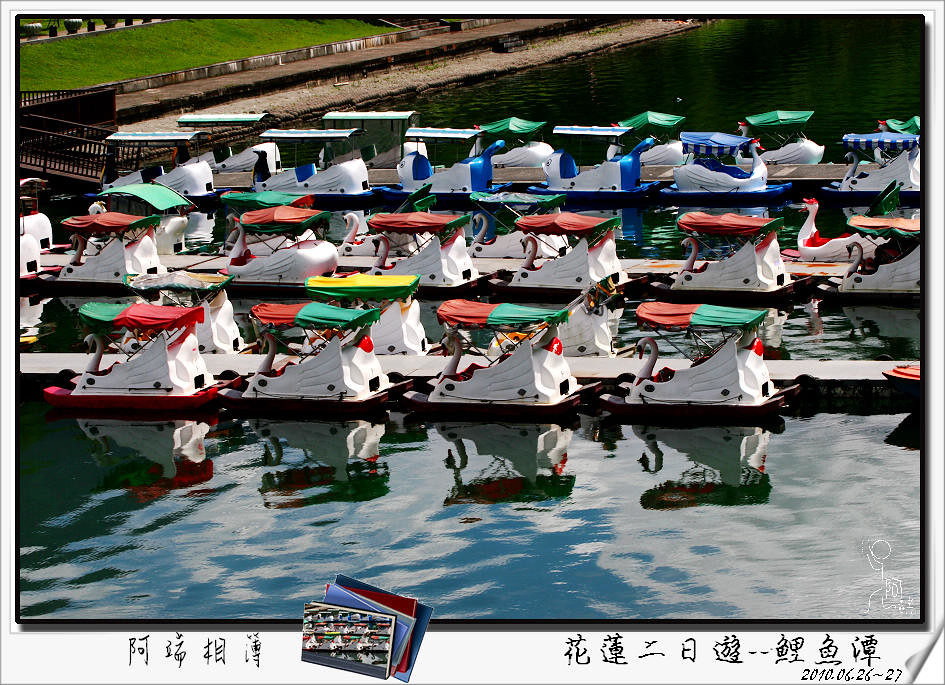The photograph depicts an overhead view of a marina featuring three rows of identical, swan-shaped pedal boats docked on shimmering blue water. Each boat has a prominent bird head—resembling a swan or goose—forming the bow, with intricately designed wings along the sides. The boats, all primarily white, have colorful tops in varying combinations of red, green, blue, and yellow. They are aligned in neat rows with water spaces in between and are anchored to a platform that runs across the scene. Towards the upper right of the image, there's an additional walkway bordered by grass. At the bottom of the photo, a white border contains black lettering in an Asian language, possibly Chinese, Japanese, or Korean, indicating the date "2010-06-26 to 27."